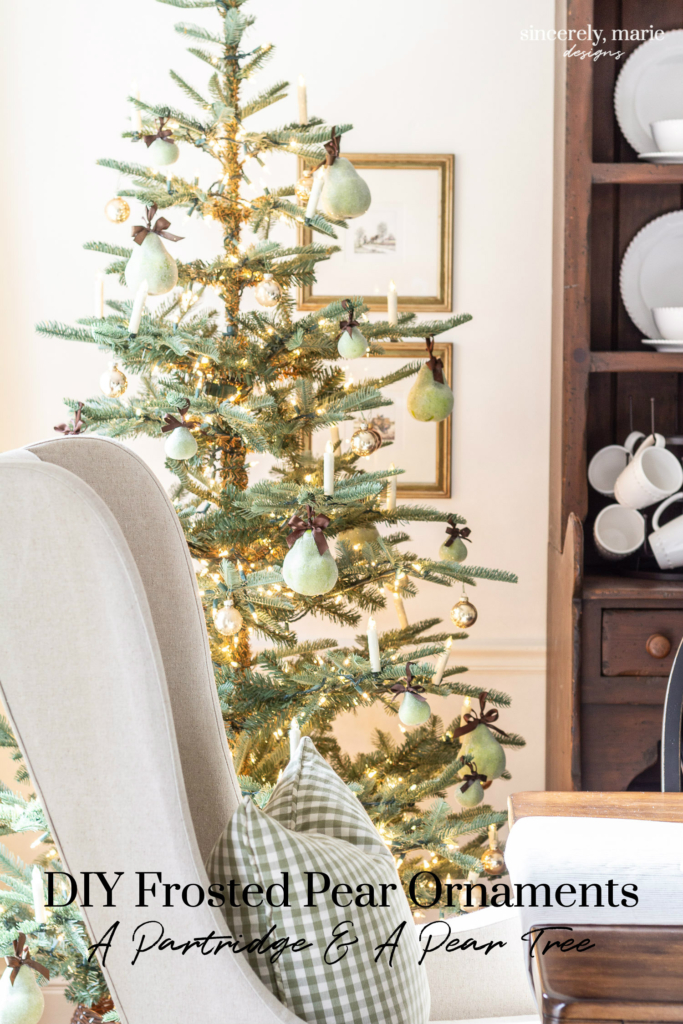The image depicts the right corner of a cozy room, featuring an advertisement for DIY frosted pear ornaments. The focal point of the scene is a sparse Charlie Brown-style Christmas tree adorned with pears of varying shades of green and white, with some lights adding a festive touch. The tree is positioned in the background, partially obscuring a few small, gold-framed pictures hanging on the wall.

To the left of the tree, a high-back wing chair, upholstered in a cream color, sits with a checkered pillow resting on it. Directly over the armchair in black letters is the text: "DIY frosted pear ornaments, a partridge and a pear tree."

On the right edge of the picture, a wooden china cabinet stands prominently. The top shelves of the cabinet display various plates, cups, and saucers, while coffee cups hang neatly from the bottom shelf. Additionally, there's a wooden table to the right of the armchair, draped with a white cloth, contributing to the warm and inviting atmosphere of the room.